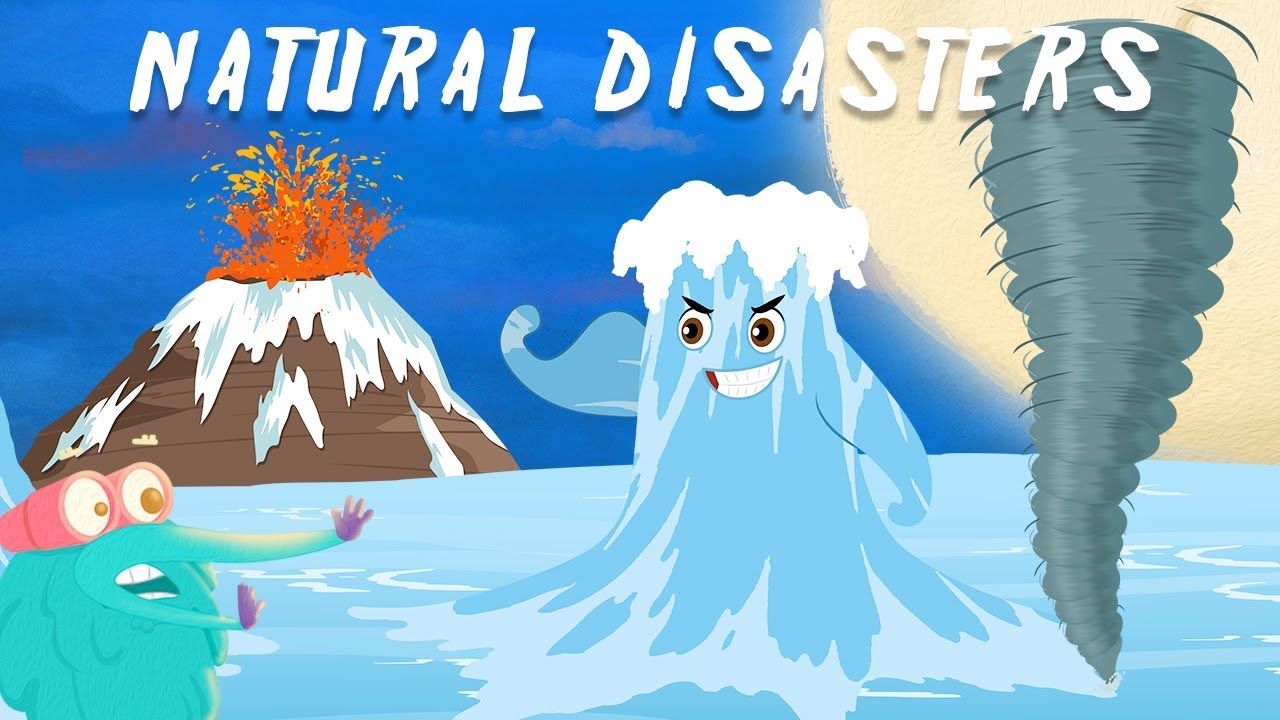The image appears to be an illustration from a child's book, titled "NATURAL DISASTERS" in bold white capital letters at the top against a backdrop of a sky with a sun or moon on the right. Dominating the scene is a playful yet menacing portrayal of various natural disasters. On the left, an erupting volcano spews lava against the sky. In the middle, a personified, muscular wave, likely representing a tsunami, rises from the ocean with a clenched fist, menacing eyes, and a sneer. To the right, a towering gray tornado swirls ominously. In the bottom left corner, a small, frightened green character with googly eyes and tiny purple hands, possibly a quirky creature, faces the disasters, adding an element of whimsy to the serious theme.